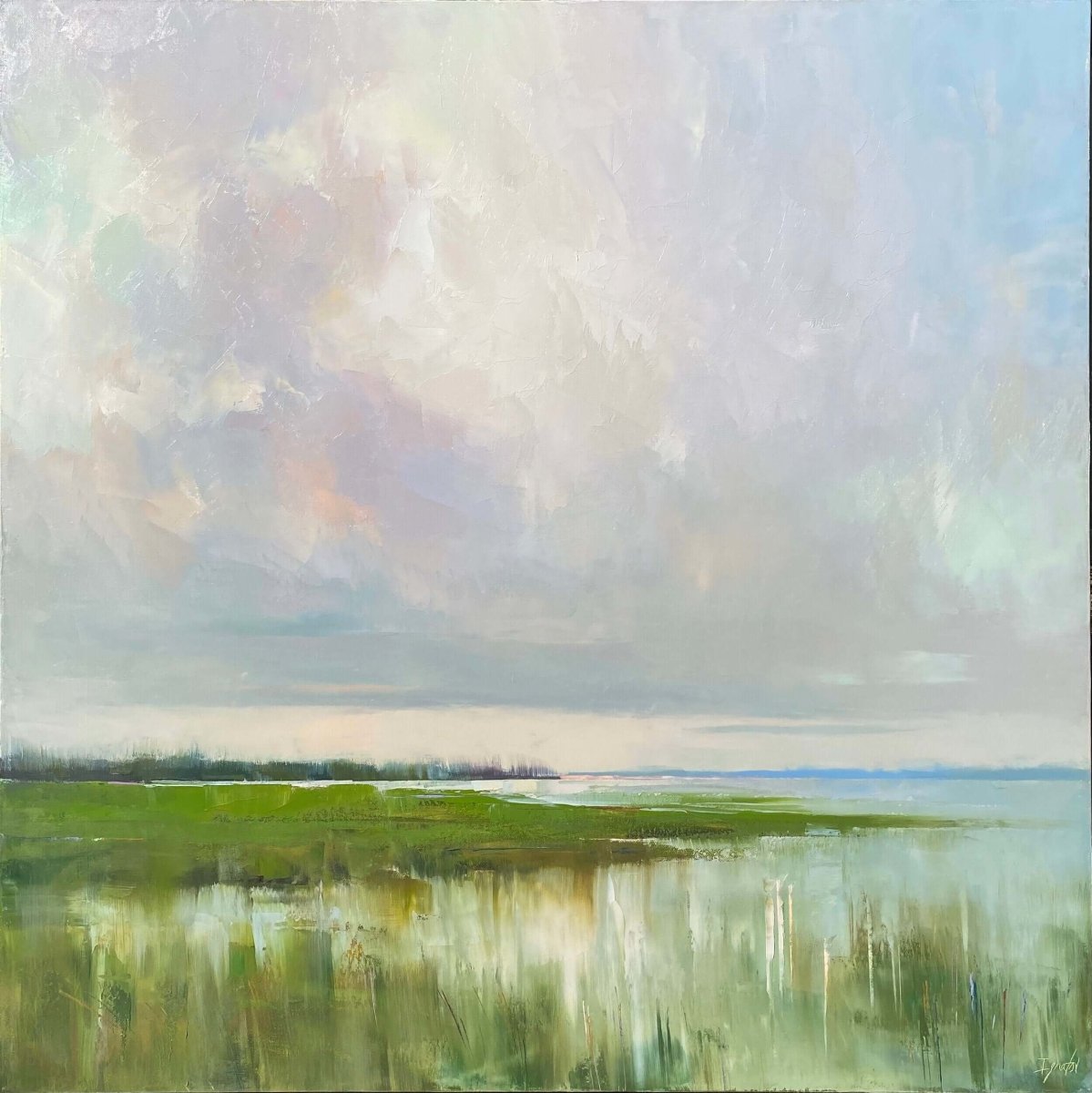This square watercolor painting depicts a serene marshy landscape. In the foreground, a body of light green-bluish water is framed by patches of green grass and plants, with some of the foliage appearing in textured paint drippings. The horizon features more greenery, creating a lush, tranquil scene. Above, the sky blends hues of white, gray, light blue, and light purple, swirling together to convey a colorful, yet overcast day. The heavy gray clouds reflect on the surface of the water, enhancing the subdued, calm atmosphere of the artwork.